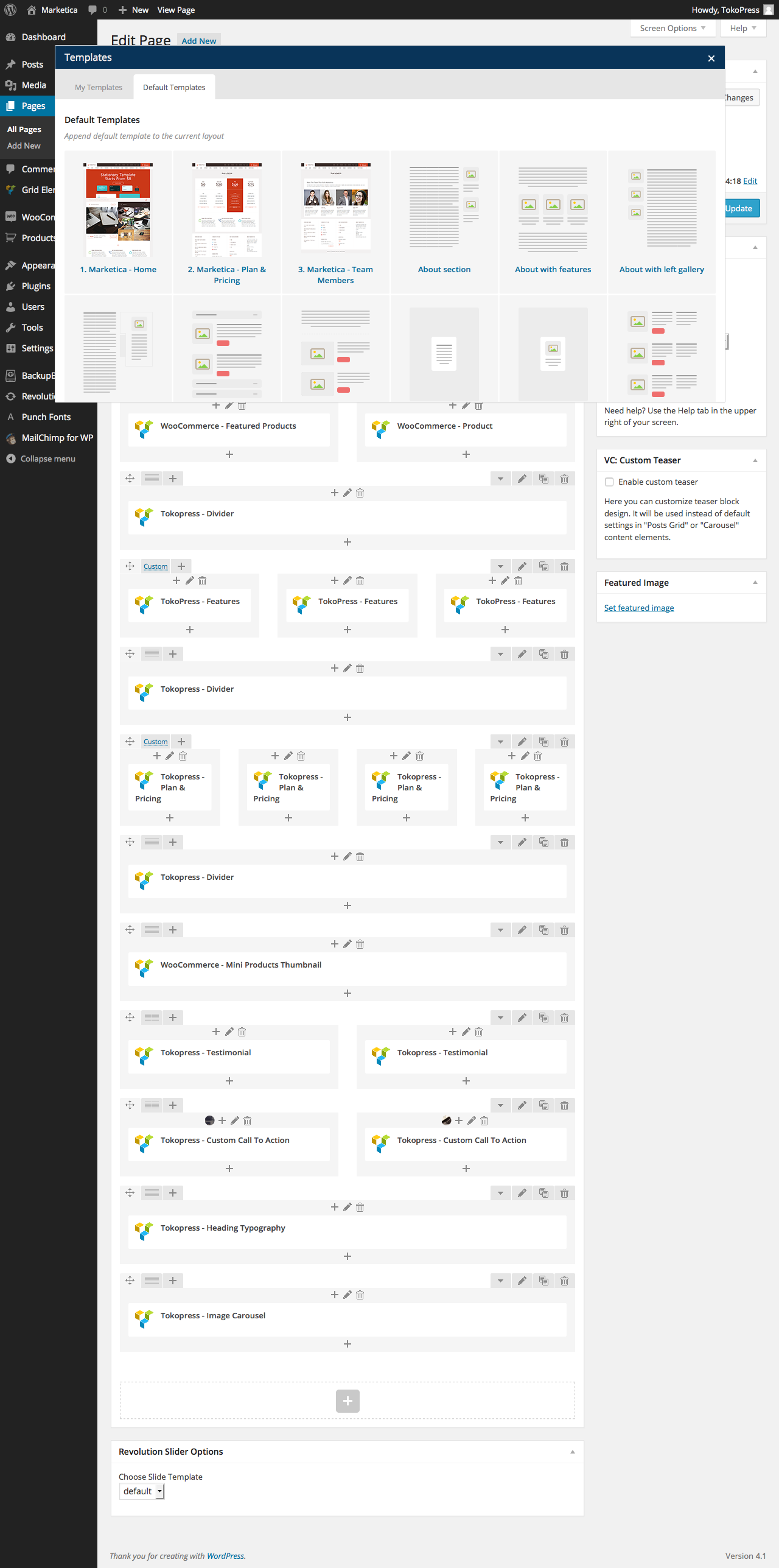The image displays a screenshot of a website interface. At the top, there is a thin, black banner featuring a home icon followed by the name "Marketica" in all capital letters: "MARKETICA". Next to it, the number zero and options for "+ New" and "View Page" are visible.

On the left side, a vertical sidebar showcases a navigation menu highlighted in a blue band. The menu includes options such as "Dashboard," "Posts," "Media," and "Pages," with the "Pages" section expanded to reveal "All Pages" and "Add New."

A pop-up banner obscures part of the sidebar, labeled "Templates". This pop-up details options like "My Templates," "Default Templates," and the ability to "Append Default Template to the Current Layout."

Further down, the image lists various sections under "Marketica," including "Marketica Home," "Marketica Plan and Pricing," "Marketica Team Members," "About Section Features," "About with Features," and "About with Left Gallery." Below these headings, a segment titled "Graphics" is shown.

The main content area features text descriptions about different features, repeatedly mentioning "Tocopress features."